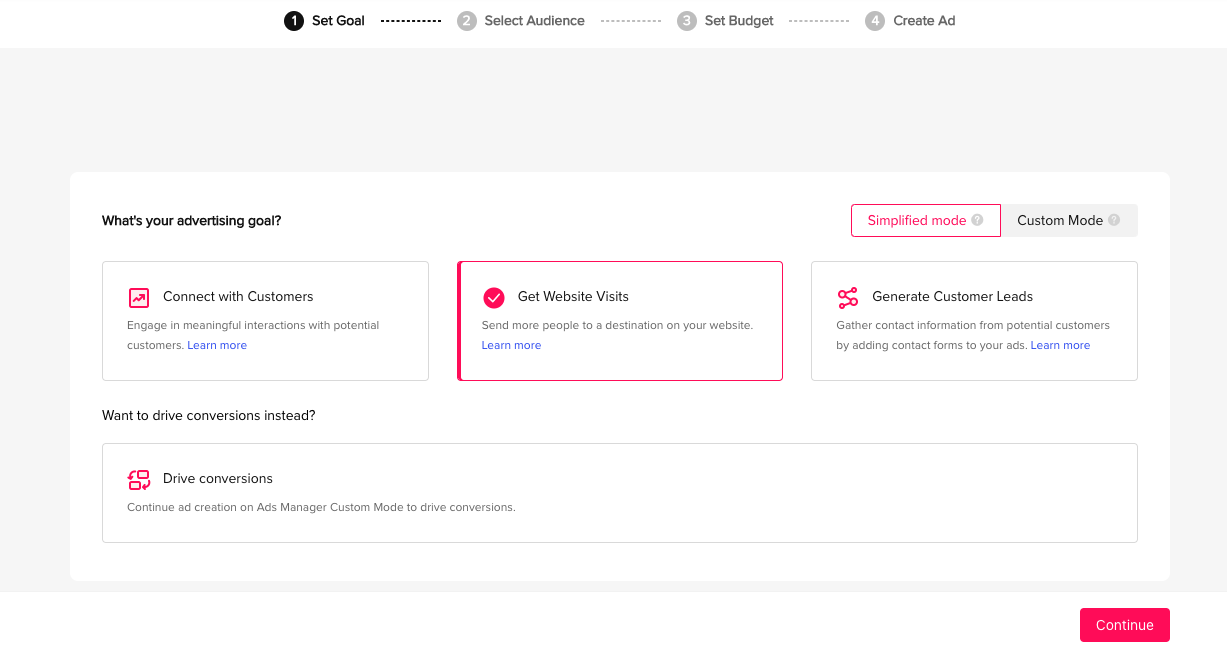This screenshot captures an ad creation interface with a predominantly gray background. Centered at the top of the image, there are four sequentially numbered steps to guide users through the ad creation process. Each step is connected by dotted lines. 

1. "Set Goal" is the first step, displayed in bold black text towards the left.
2. Moving rightwards, connected by a row of horizontal dots, is "Select Audience" shown in gray.
3. Similarly connected by another row of dots, the third step is "Set Budget," also in gray.
4. Finally, the fourth step, "Create Ad," is presented in gray.

Below these steps lies a large white box, part of the expansive gray background. This box is where users can set their advertising goal. On the top left of this section, in smaller black letters, is the prompt "What's Your Advertising Goal?" Below this prompt, three goal options are available in distinct boxes:

- The first option, "Connect with Customers," includes a brief description underneath.
- The middle option, "Get Website Visits," is highlighted in red, indicating it is currently selected.
- The third option, "Generate Customer Leads," sits to the right.

Towards the bottom left of the white box, there's a prompt in small black letters stating, "Want to Drive Conversions Instead?" Underneath this prompt, a large horizontal column labeled "Drive Conversions" is displayed. At the bottom right corner outside the gray box, there's a prominent red button labeled "Continue," inviting the user to proceed to the next step.